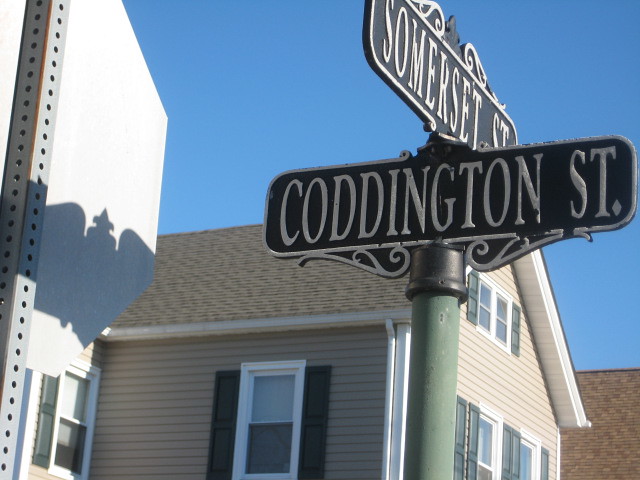The image captures a slightly upward view of street signs mounted on a tall, bluish-gray pole with a darker gray cap. Central to the image is a black street sign with a silver border that reads "Coddington St." in silver text, positioned horizontally. Above it, there is another sign for "Somerset St." angled diagonally from the top left down to the right. Both signs have a similar design. In the background, against a blue sky, a gray-sided house with white trim and green shutters is visible. The house features multiple windows, including a prominent attic window and several regular windows. To the right of the primary house, a rooftop with brown shingles from another house is partially visible. On the left side of the image, the back of a street sign, likely a stop sign, is seen with its supporting metal rod running vertically along the side.